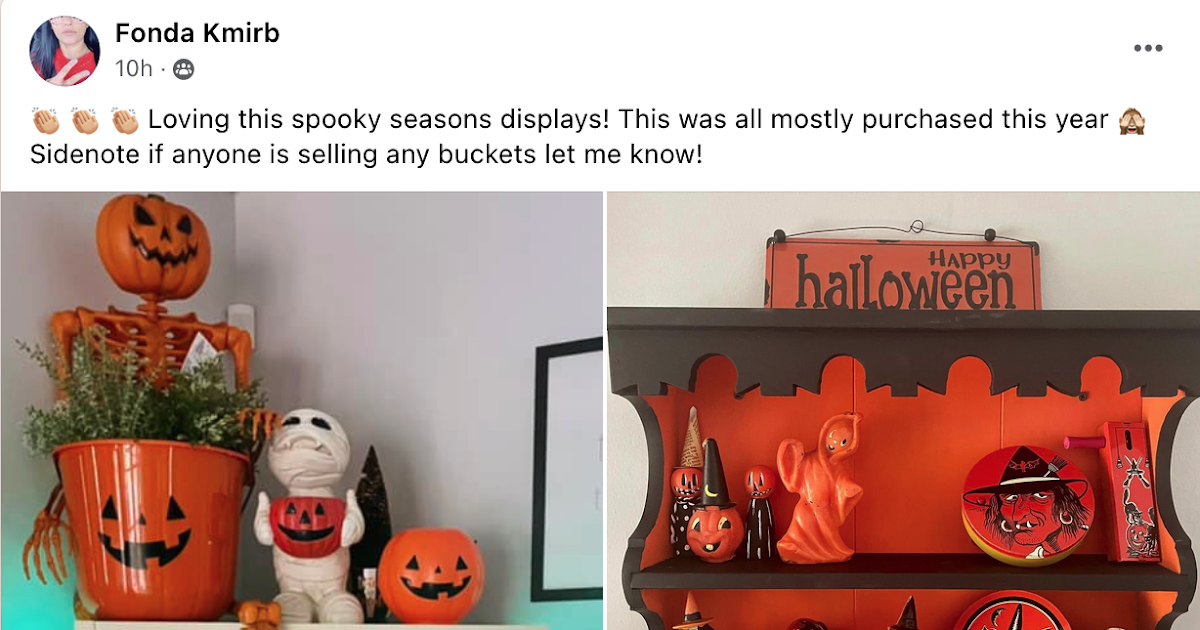This image showcases a detailed scene of Halloween-themed displays. At the top, a computer screen is visible. On the left side of the screen, there is a circular image of a woman with dark hair framing her face. Her eyes are not visible in the shot, but her nose, mouth, and part of her chest are. She is wearing an orange shirt and has two raised fingers resting against her chest. Next to this circle, a label reads "Fonda KONDA" with the last name "KMIRB" followed by "10-H". Below this, there are three hand clapping emojis with the text, "Loving this spooky season's displays! Most of these were purchased this year. Side note, if anyone is selling any buckets, let me know!"

Beneath the text, there are two side-by-side images. The left image displays a beige wall in the background. In the corner, there is an orange skeleton with a pumpkin head and a pumpkin basket filled with greenery underneath it. Both the skeleton and the pumpkin have black eyes, noses, and mouths. Next to these, there is another skeleton figure, also with a pumpkin head featuring the same jack-o-lantern face, and a pumpkin bucket below it with matching black features.

The right image also features a beige background wall. A wooden shelf is visible with an orange Halloween sign on top that reads "Happy Halloween." Below this sign are various decorations, including pumpkins adorned with witch hats, a witch figure on the left side, and another circular display with an orange face and a witch’s hat.